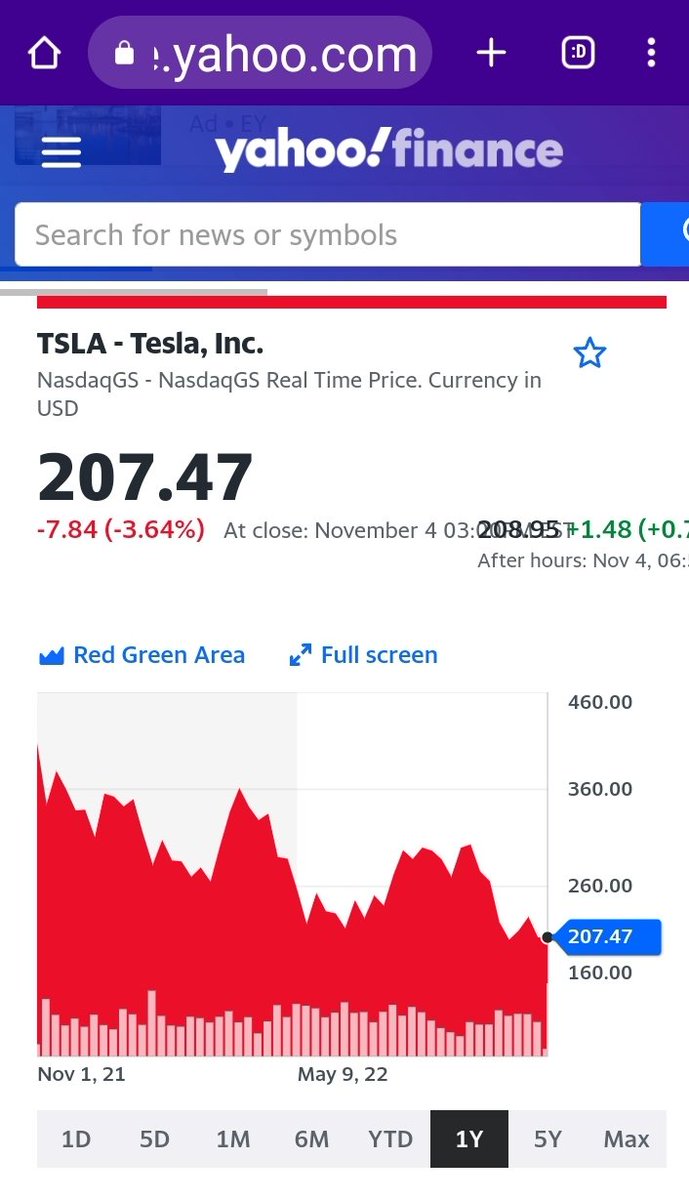This image is a screenshot from the Yahoo Finance website, displaying a detailed view of Tesla Inc.'s (TSLA) stock index. At the top, the stock symbol, "TSLA," is accompanied by the company's name, "Tesla Inc.," and its listing on NASDAQ GS, with real-time pricing in USD. The central focus shows the stock price at $207.47, reflecting a decrease of $7.84 or 3.6% as of the market close on November 4th. The screenshot also includes after-hours trading details for the same date.

The chart within the image has an L-shaped scale. The vertical axis on the left ranges from 160 to 460, specifically marking values such as 160, 207.47, 260, 360, and 460. The horizontal axis at the bottom displays a time-lapse from November 1st, 2021, to May 9th, 2022. The price point of $207.47 is prominently highlighted within the chart. The overall layout of the screenshot is rectangular.